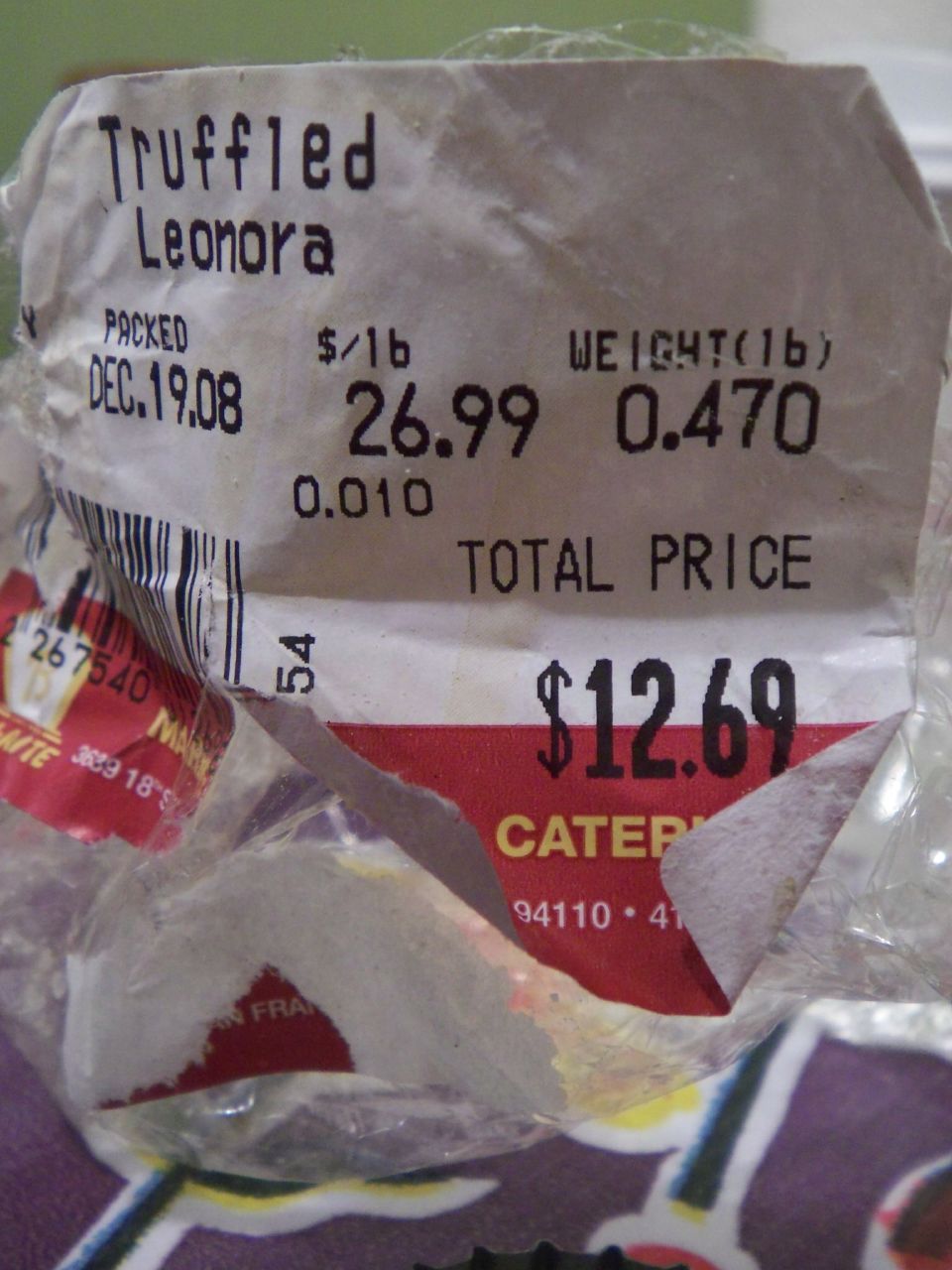The image depicts a slightly crinkled, predominantly white food tag. In the top left corner, the tag is labeled "Truffle Lenora" in black regular font. Just below and to the left, the tag notes the packing date as "Packed December 9th, 2008" and includes "12.09.08". Slightly to the right, the price per pound is listed as "$26.99". Beneath the price per pound and slightly to the left, the weight is marked as "LB 0.470". Directly below the $26.99, there's a smaller printed number, "0.010". To the left of this information, there's a barcode. Adjacent to the barcode, the total price is displayed as "$12.69". The tag also features a red section on the lower part, though it is torn, making some text and numbers illegible.